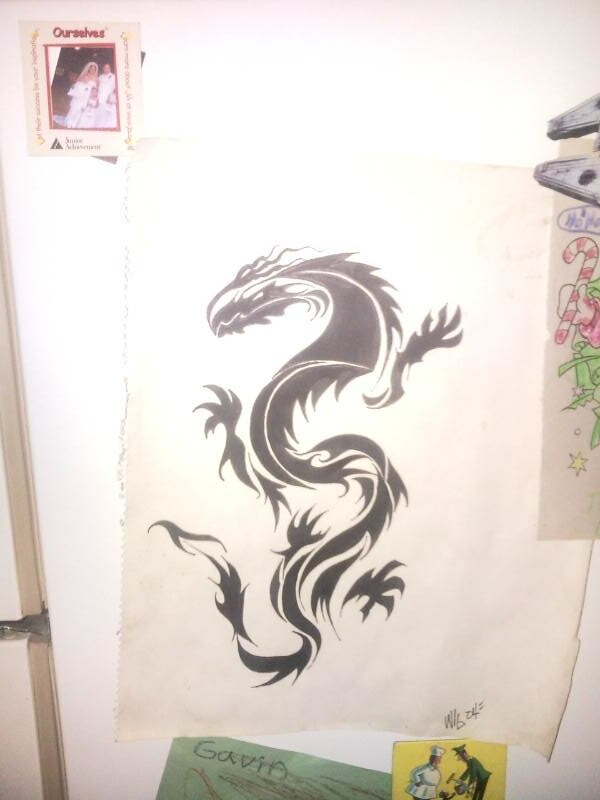This full-color photograph appears to have been taken in Warsaw and features a rectangular image set against a predominantly white background. Dominating the center is a detailed black dragon drawing, characterized by its long, winding tail and intricate hands and feet resembling tentacles. The dragon's head is pointed towards the lower left.

The photograph includes several additional elements: 

- In the upper left-hand corner, there's a small wedding photo with a white background and a red printed frame. 
- On the far right, a hand-drawn candy cane can be seen, although the border cuts off part of the candy cane and other potential decorative items. 
- At the very bottom, there's a green cloth with the handwritten word "Gavio." Next to this cloth, a yellow piece of fabric features a small image of two men—one dressed in a baker's uniform with a white cap and the other in a brown cap, possibly a police officer.

Red lettering saying "ourselves" appears prominently near the wedding photo. The entire composition is framed with a red border, bringing all these diverse elements together into a cohesive and captivating visual narrative.